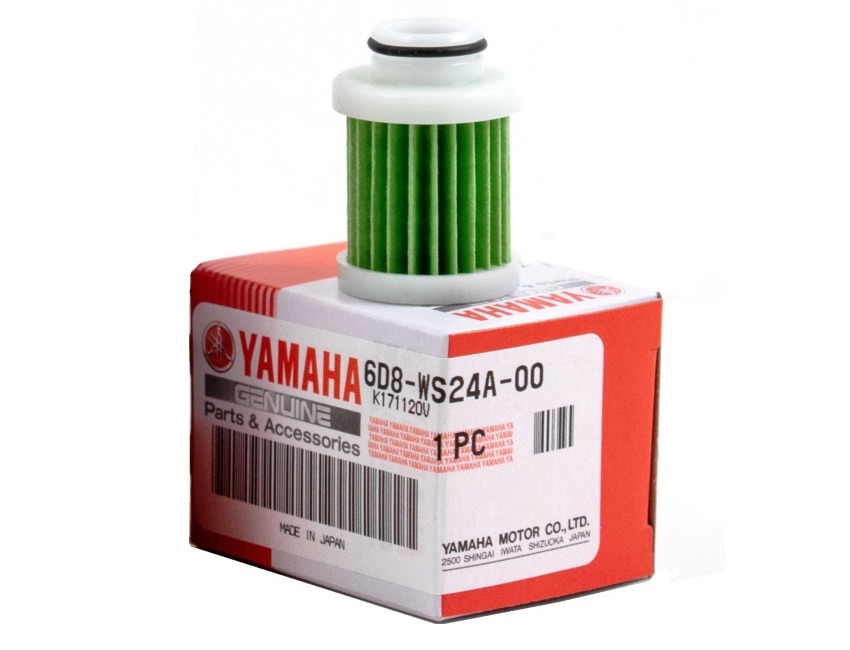The image displays a close-up of a Yamaha parts and accessories product. At the bottom of the image, there is a red and white cardboard box with the Yamaha logo prominently displayed in red font. Below the logo, the text reads "genuine parts and accessories," and there is a black and white barcode along with a note stating the product is made in Japan. Additional details like part number information and an indication that there is one piece inside the box are also visible.

On top of the box, there is a green filter, likely intended for a car or motorcycle. This filter has a cylindrical shape with two white plastic caps on the top and bottom, and the primary filtering material is green, pleated paper. The filter has green fins and includes a small rubber ring at the top, suggesting it attaches securely to another component. The entire scene is photographed against a white background from a side perspective.